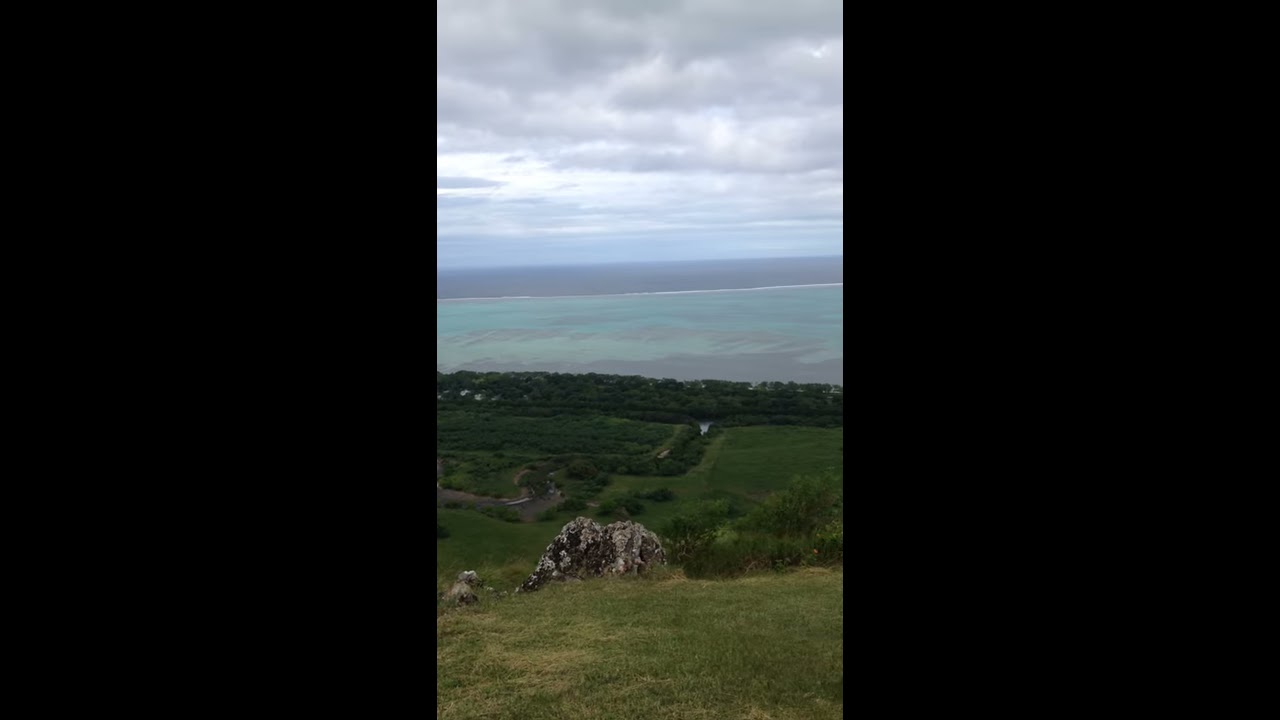This vertical photo, taken outdoors, prominently features a landscape view from an elevated hill or cliff. The image is uniquely segmented into three equal parts: both the left and right segments are solid black, while the central segment showcases the natural scenery. In the foreground, the hillside is adorned with green grass, various vegetation including bushes, and several rocks and rounded boulders. The lighter green grass suggests the area is well-lit, even though the sky above is a mix of overcast light and medium gray clouds. Despite the cloud cover, sunlight is streaming through gaps, casting light onto the scene below. 

The middle of the photo reveals a coastline with light blue waters transitioning into a darker blue further out, indicative of waves breaking on a distant sandbar or coral reef, creating a lagoon-like appearance. There's an observable road or creek snaking through the landscape below, and the horizon stretches out to the ocean where white-crested waves are visible. Amidst the natural splendor, a few trees emerge from the hillside, adding to the serene and slightly wild ambiance of the scene.